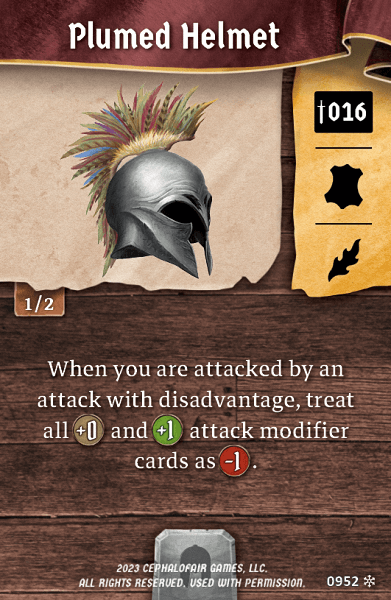The image features an intricate, detailed design. At the top, there is a band showcasing various shades of brown, including two darker shades, transitioning into a burgundy color. Beneath this band, a gold outline frames the section. On the left side, there is a beige rectangle with light brown spots, resembling a camel color. Adjacent to this, there is a silver helmet adorned with numerous feathers. The feathers display a rich palette of colors, including brown, beige, green, yellow, and blue.

To the right, another rectangle appears, this one in a yellowish hue. Above this, a black rectangle contains a white sword, and within this rectangle, "016" is inscribed. A black line runs below, leading to a black shield-like shape, followed by another black line. Below these elements, there seems to be a black shape that could be interpreted as either a leaf or a flame.

The background at the bottom is composed of brown wood, overlaid with white text. The text reads: "When you are attacked" with a capital "W" for "When." The subsequent lines continue with, "by and," "attack with disadvantage," followed by, "treat or." There is an olive-colored circle with "+1" and "0" written in white inside it, and then another green circle with "+1" in white inside it. Beneath, the text reads "Attack modifier" followed by "cards as." Next, there is a red circle with "-1" written in white inside it, ending with a period.

At the bottom of the image, there is copyright information in white text: "2023 Cephalofair Games, LLC. All rights reserved. Use with permission." In the lower right-hand corner, the numbers "0952" are displayed in white, alongside a snowflake symbol.